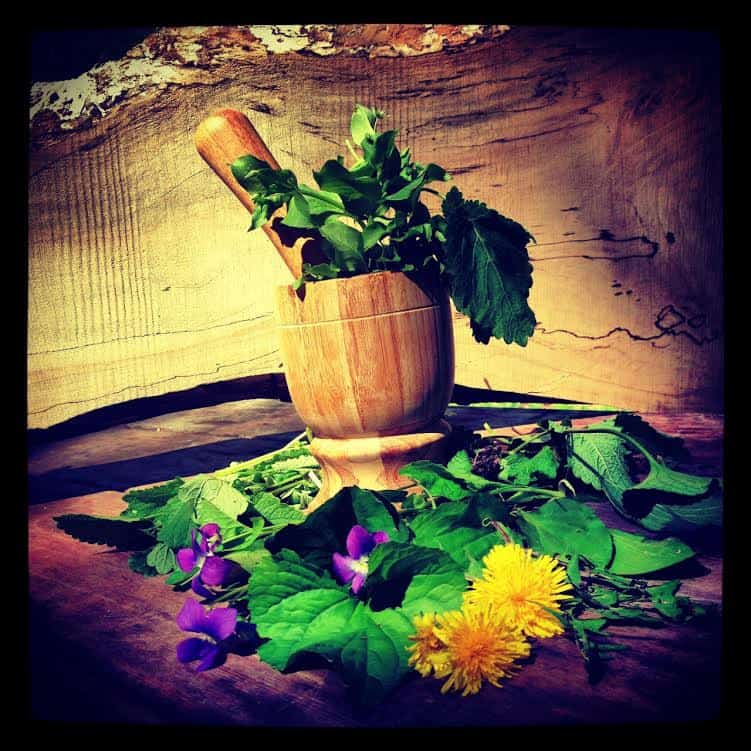The image features a side view of a light yellow wooden mortar and pestle resting on a wooden table. Inside the mortar are a variety of green plants, which could be herbs, along with the pestle itself. Surrounding the mortar at its base are additional plants, predominantly green leaves, interspersed with vibrant yellow dandelion-like shapes and a few purple flowers. The backdrop is dominated by a rugged stone wall, displaying rough, hewn shapes, which adds a rustic charm to the scene. This combination of wooden and botanical elements, set against the textured stone background, creates a natural, earthy composition.